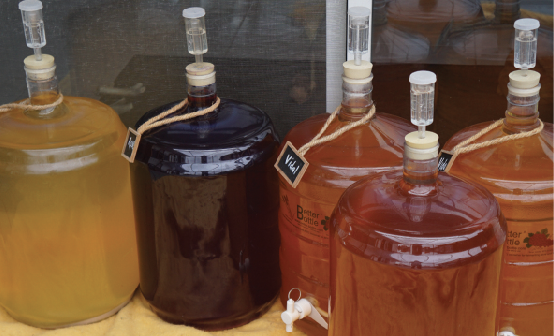This image features five large, jug-like containers, reminiscent of office water cooler bottles, each equipped with a spigot at the bottom for dispensing liquids. The jugs are topped with white plugs and a specialized apparatus resembling a syringe or needle, possibly for regulating pressure. Tied around the neck of each jug are brown strings with small signs, one of which may say "vital," possibly indicating a fruit in another language. From left to right, the liquids inside the jugs display a spectrum of vibrant colors: the first jug contains a bright yellow liquid, the next is filled with a dark purple substance, followed by a jug with a dark brown, honey-like liquid. The last two jugs both contain a similar dark brown liquid. The background of the image reveals a glass window pane, providing a clear backdrop to the foreground of colorful jugs. On the left, a yellow tail of what the jugs are sitting on is just visible. This setup appears to be involved in the production of various colorful beverages, potentially fruit-based alcohols.